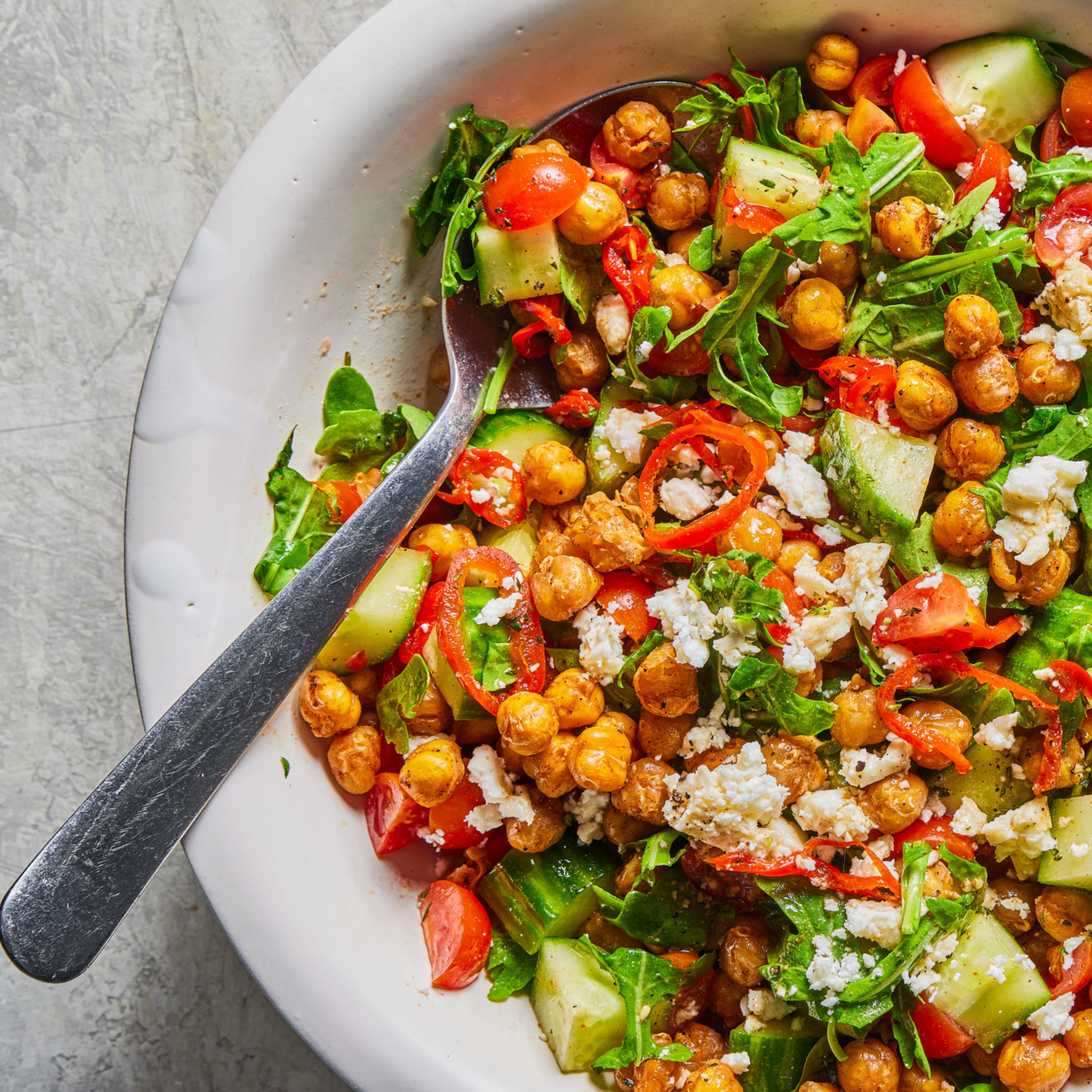The image features a vibrant and appetizing vegetarian salad served in a white bowl, set against a white marble or granite surface. The salad comprises a colorful mix of cherry tomatoes, garbanzo beans, zucchini, sliced red bell peppers, and what appears to be arugula or possibly spinach. Scattered among these ingredients are chunks of feta cheese, adding a creamy texture. There's a sprinkling of salt and pepper, and possibly some shaved parmesan providing an additional layer of flavor. A silver serving spoon is placed on the left side of the bowl, with its handle visible above the food. The photograph captures about two-thirds of the bowl from a top-down, close-up angle, making the textures and colors of the fresh ingredients really stand out.